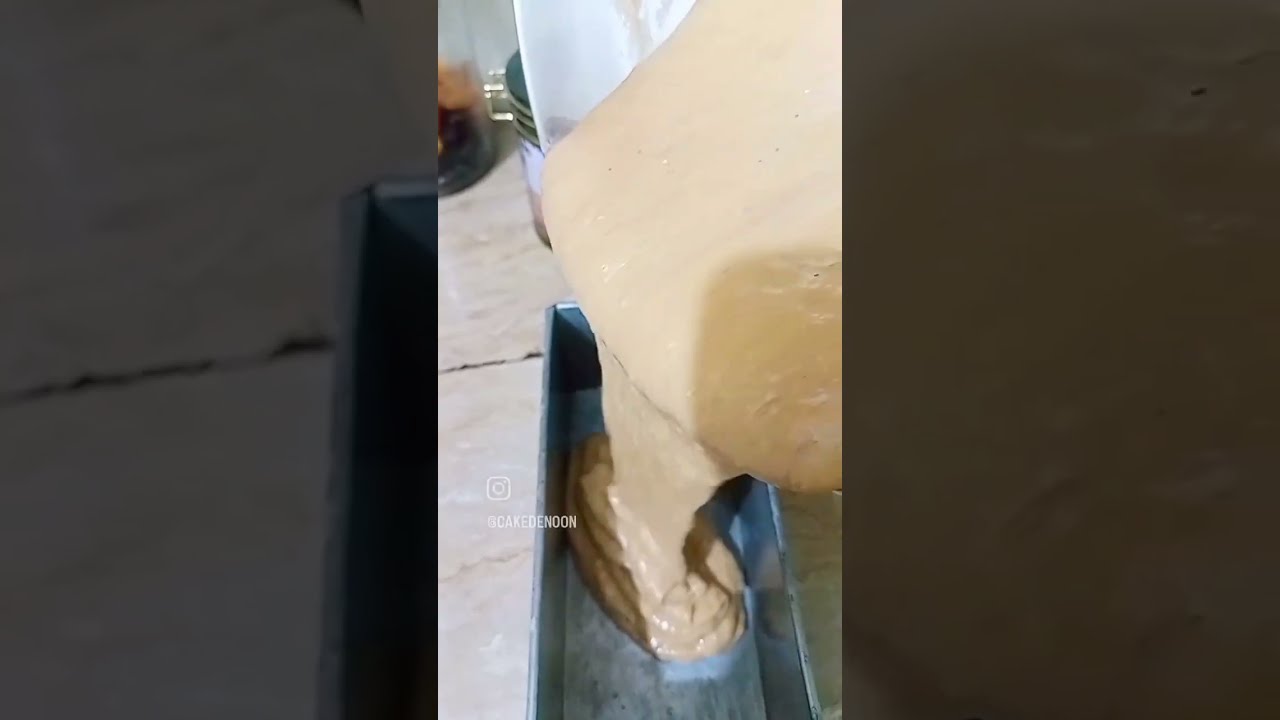The image prominently features the act of pouring a thick, light yellowish-tan batter from a white or silver bowl into a metallic gray rectangular baking pan. The setting appears to be on a brown table, possibly wooden, with visible lines suggesting the seams between wooden planks. In the background, there are some jarred ingredients and a glass containing a reddish drink. The left and right edges of the image are zoomed-in, darker close-ups of the main image, showcasing detailed textures of the table and the substance being poured. Within the central part of the frame, a tiny caption in white text hints at the words "SS cake DE noon," though it’s almost unreadable due to its size. The scene suggests someone is in the process of baking, likely preparing a dessert or bread.